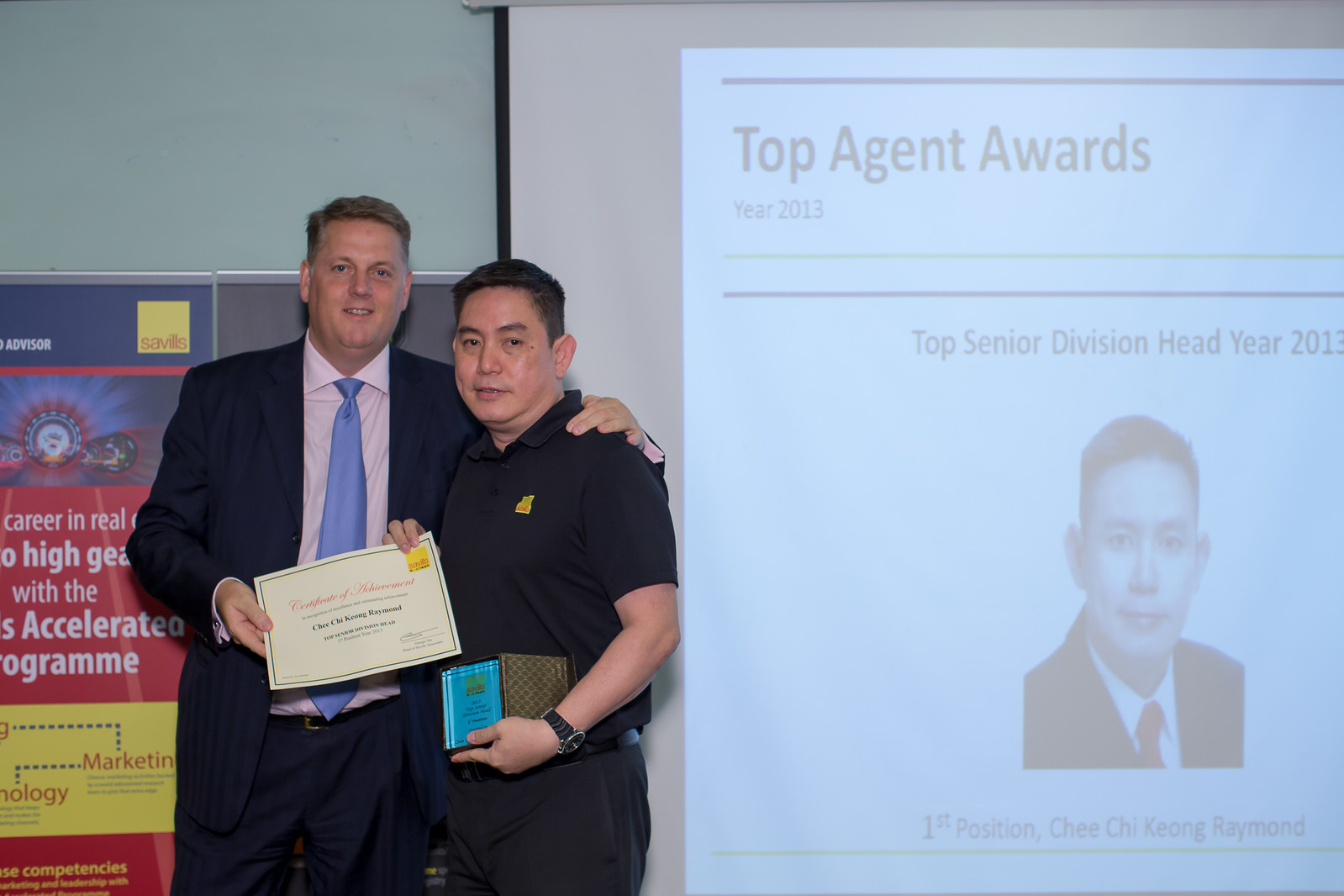In this indoor photograph, we witness a celebratory moment at an awards ceremony. The image, taken in landscape mode, features a rectangular screen on the right-hand side displaying a blue projection. The projection reads "Top Agent Awards Year 2013" in light gray at the top. Below, it states "Top Senior Division Head Year 2013," and features a headshot of an Asian man, identified as "First Position Chi Chai Kyong Raymond." 

In the left-center of the image, we see two men facing the camera. The individual on the right matches the image on the projector; he is an Asian man with short-cropped black hair and light brown skin, wearing a black polo shirt with a yellow emblem and black slacks. He holds a blue award plaque in his left hand and grasps the corner of a certificate in his right.

Next to him stands a taller Caucasian man in a navy blue pinstriped dress jacket, light pink collared shirt, and blue tie. The Caucasian man holds the other end of the certificate and has his left arm affectionately draped over Raymond's shoulders. Behind them, on the left, a green-bordered wall is partially visible, adorned with a banner advertising career goals, though the text is obscured.

The predominant colors in the image include various shades of gray, blue, silver, red, light blue, yellow, tan, and black. The setting and attire suggest a formal indoor awards ceremony.